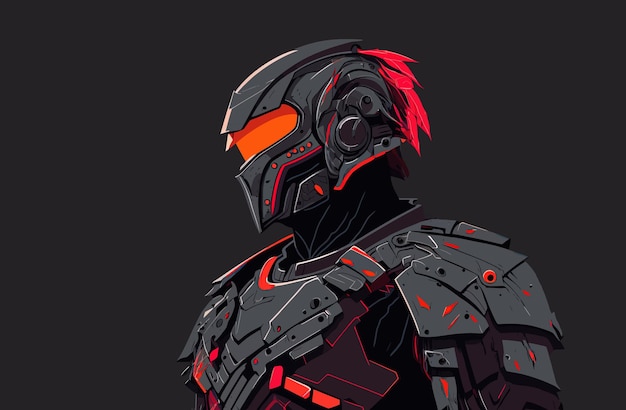This detailed illustration depicts a character evocative of the Halo franchise, clad in a highly advanced exoskeleton suit. The armor, predominantly steel gray and black, is sharply detailed with strategic highlights in neon flame red, flame orange, and pink accents, giving it a vibrant and dynamic appearance. Angular shoulder pads, an intricately designed helmet, and multiple metallic plates characterize the suit. The helmet's visor is a striking orange, completely obscuring the individual's eyes, with pink lines and buttons adorning its surface. Notably, a tuft of pink or red feathers extends from the back of the helmet, adding a unique flair. Additional pink squares and buttons are interspersed across the armor, complemented by dark purple plates situated beneath the primary gray and black sections. The image is framed against a uniformly dark gray background, showcasing the character from the head to just about mid-chest level in a slightly angled, left-facing stance.